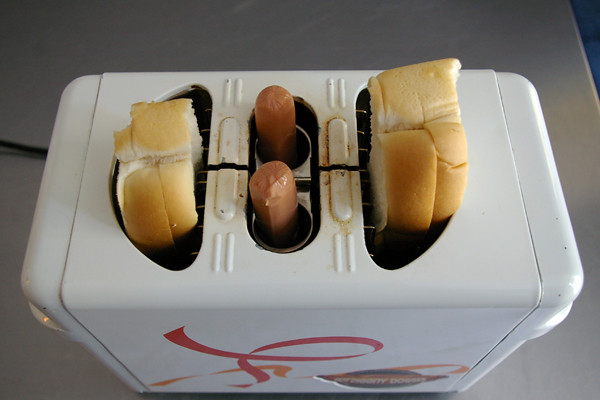In the image, we see a white multifunctional kitchen appliance designed to both toast bread and cook hot dogs simultaneously. The device features three main slots: the left and right slots, which can hold slices of bread or hot dog buns, and the middle slot that is divided into two circular holes for placing hot dogs. The bread in the left and right slots appears to be thick slices of white bread, possibly Texas toast or French bread, while the middle slot visibly holds two uncooked hot dogs. A distinctive red and orange swirl design or logo is present on the side of the appliance, although it becomes blurry upon zooming. Additionally, there is a black power cord located at the upper left-hand corner. The entire setup is situated on a light gray, possibly slate, countertop, emphasizing the appliance's pristine and functional design.